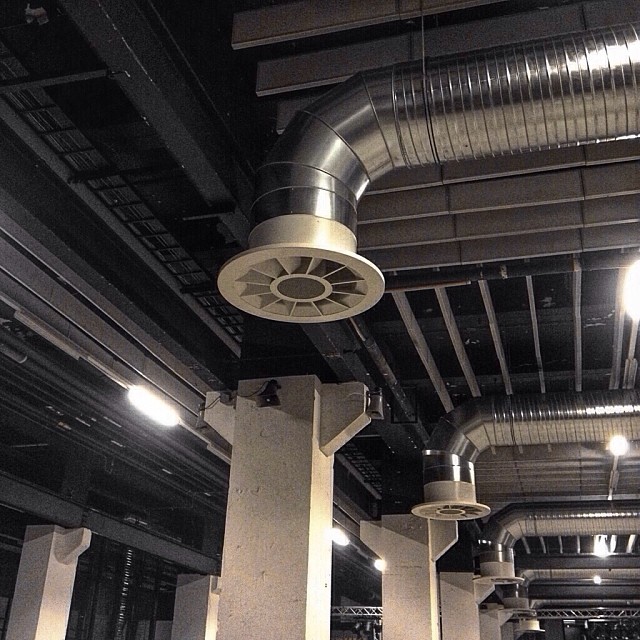This photograph captures the interior ceiling of a large industrial facility, prominently featuring an intricate network of modern, shiny ductwork likely used for air conditioning or heating. The metallic ceiling beams are interspersed with large corrugated aluminum ducts, each equipped with an elbow joint leading to a beige, fan-like end piece. The ducts appear to fade into the distance, highlighting the vast expanse of the space. Supporting this high, largely black ceiling are two rows of tall, light gray or possibly white concrete columns. These columns and ducts together reveal the exposed structural elements of the building, contributing to its stark, industrial aesthetic. The image, rendered in black and white, emphasizes the contrast between the dark ceiling and the lighter support columns.